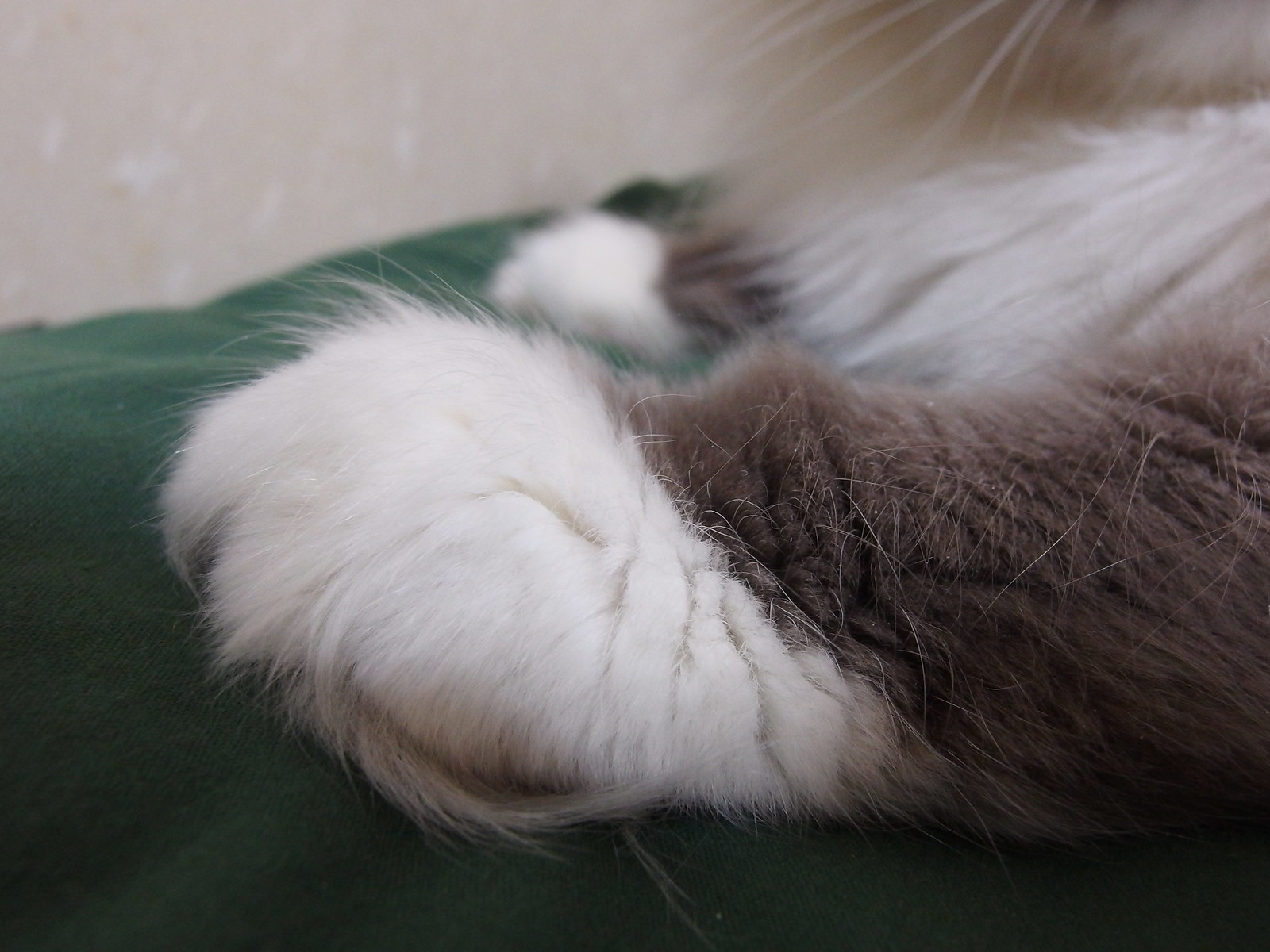This color photograph presents a close-up, side view of a cat's front left paws. Both paws are featured, with the tips covered in thick white fur, which extends into long strands curling back from the bottom. The legs above these paws are dark gray, transitioning into a charcoal hue. The image captures intricate details, including individual hairs on the fur, and hints at the cat's body, showing a portion of its white chest fur and some white whiskers emerging from the upper right. The backdrop shows a slightly blurred off-white or creamy gray background, likely a couch or wall. The cat is comfortably resting on a hunter green blanket, adding a rich contrast to the detailed gray and white fur.